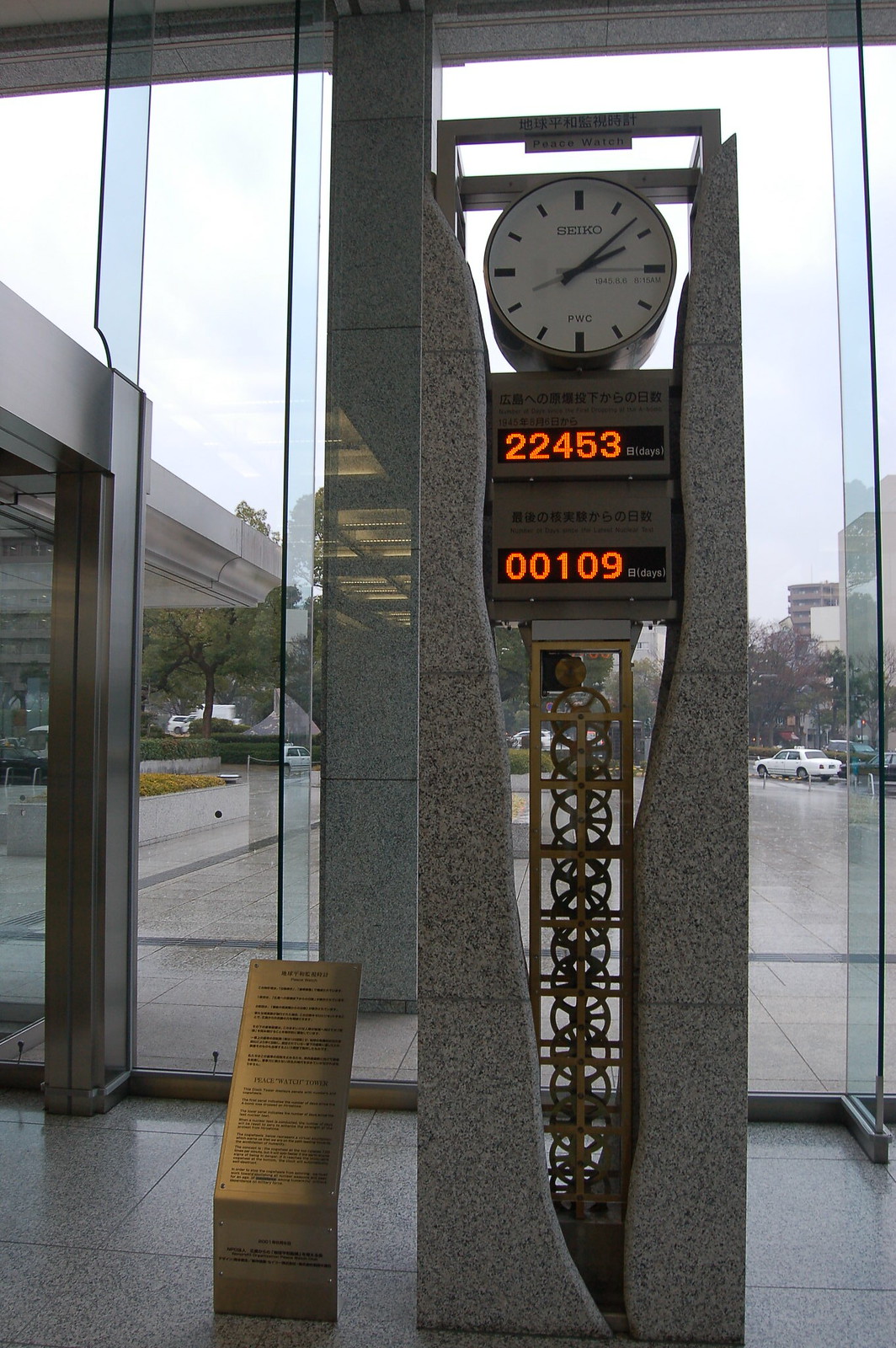In this image, a striking clock is prominently displayed at the entrance of a modern building characterized by its glass walls and door, enhanced by various metal outcroppings and panels. The exterior scene reveals wet stone walkways and a few parked cars, suggesting recent or ongoing rain. Inside, a grand stone installation houses the clock, which features digital countdown displays in bright red font at the bottom. To the left of the clock, a metal sign provides detailed information about the sculpture, adding to the sophisticated ambiance of the space.